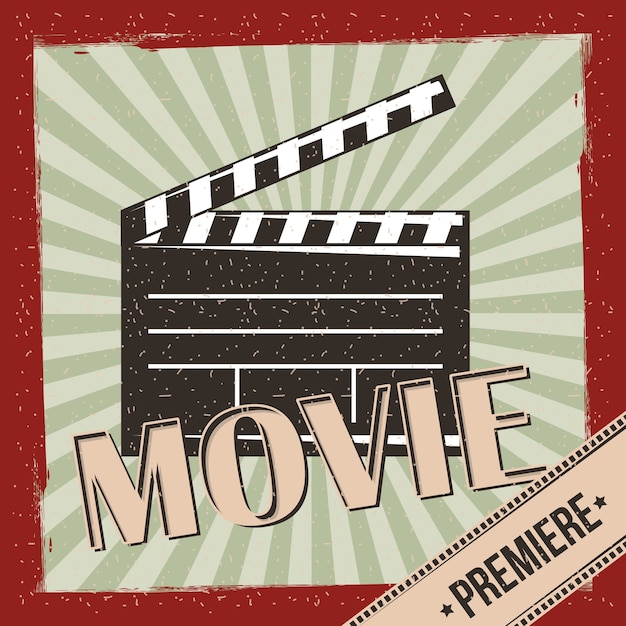This image is an advertisement poster for a movie premiere, featuring a distressed red border with white speckles. In the center, it showcases a radiating sunburst design in varying shades of green—alternating between light and slightly darker hues. Dominating the middle is a black and white movie clapperboard, commonly used to signal action during filming. Across the clapperboard, in large tan capital letters, is the word "MOVIE." Positioned diagonally at the bottom right corner is a banner resembling a strip of film, complete with black dots along the top and bottom edges. This banner, adorned with stars on either side, prominently displays the word "PREMIERE" in distressed black lettering, emphasizing the occasion of the movie premiere. The overall layout is simple yet evocative, evoking the aesthetics of classic film industry motifs.